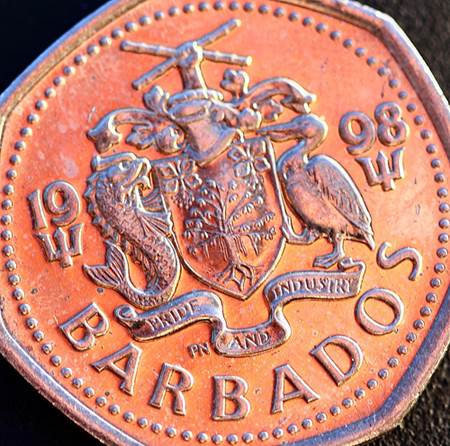This color photograph, presented in a square format, showcases a coin with a copper-orange hue displayed against a black background. The coin's rim is silver with an irregular outline, and there are raised silver dots around the inner edge. The coin, though not perfectly round, appears slightly misshapen and has a raised edge. Taking up the majority of the picture, the top, bottom, left, and right sides of the coin are cut off by the picture's edges.

In the center of the coin, a detailed shield is depicted. The shield displays two flowers in the upper left and right corners with a tree below them. To the left of the shield, there is a curled fish, and to the right, a bird resembling a heron or crane. Above the shield, there is what appears to be a piece of armor with a raised fist and crossed bars. Beneath the shield, a banner reads "Pride and Industry."

On either side of the shield, the numbers "19" and "98" indicate the coin is from the year 1998, each number positioned above a trident symbol. Around the bottom edge of the coin's circle, the word "BARBADOS" is prominently displayed in raised letters. The coin is a striking representation of Barbados' pride and industry, captured in a rich, photographic realism style.